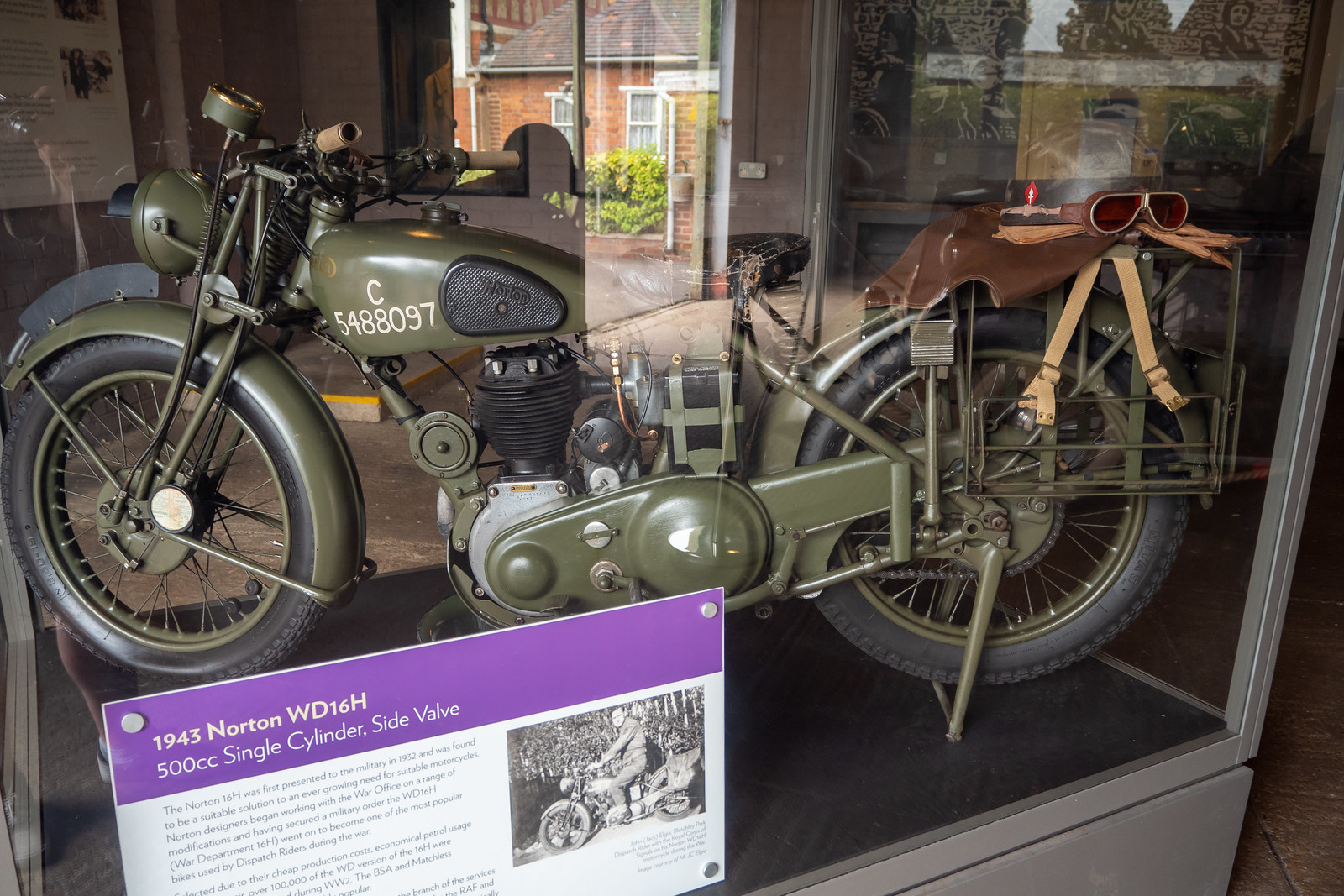This image captures a detailed display at a museum featuring a meticulously preserved, old military-green 1943 Norton WD16H motorcycle. Encased in glass and elevated on a platform, the motorcycle faces towards the left, revealing intricate details. Distinguished by its army-green color, the motorcycle sports a leather-strapped brown bag over the back wheel and a pair of red riding goggles. The identification "C5488097" is prominently displayed in white text between the handlebars and the seat. Accompanying the exhibit is an informative plaque at the bottom of the glass case, marked by a purple bar and white text that reads, "1943 Norton WD16H, 500cc single cylinder side valve." An adjacent photograph shows the motorcycle in action during its era, complemented by descriptive text providing historical context.